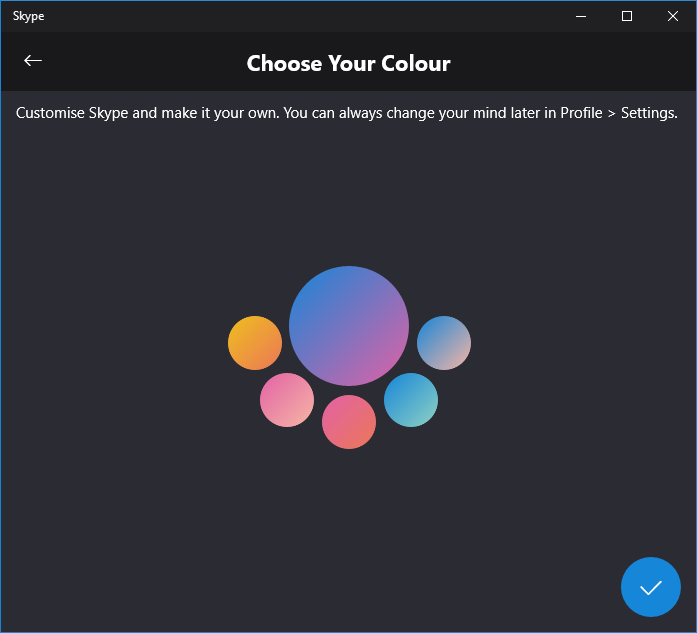This image features the interface of the Skype application, not a web page. In the top left corner, the Skype logo is prominently displayed. The top right corner houses the typical window controls, including the minimize, maximize, and close buttons. The main content area presents a customization prompt with the text: "Choose your color. Customize Skype and make it your own. You can always change your mind later in the profile settings." Below this text, there is a color selection array featuring hues of orange, lavender, pink, and blue, each displaying shifting gradients. The background of the interface is black. Notably, a blue check mark is positioned at the bottom right corner, indicating the currently selected option or confirming a selection.